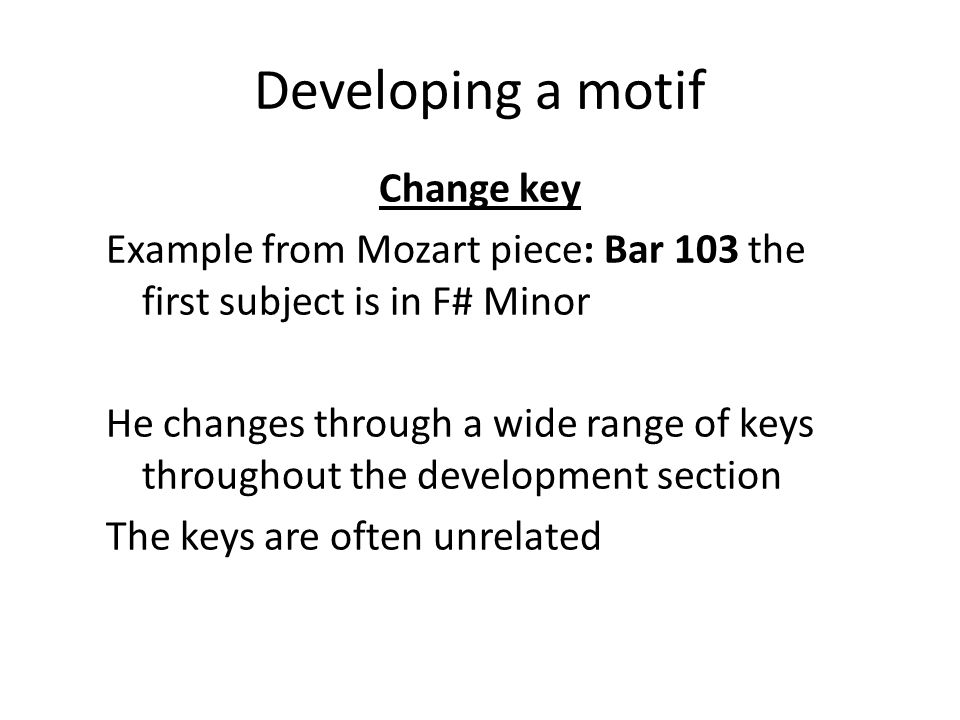The image is a slide from a PowerPoint presentation with a plain white background and black text. At the very top, the title reads "Developing a Motif." Below the title, in bold and underlined text, it says "Change Key." Following this, another line reads "Example from Mozart piece: Bar 103." Further down, it states, “The first subject is in F minor.” This is followed by a sequence of statements: "He changes through a wide range of keys," "Throughout the development section," and "The keys are often unrelated."